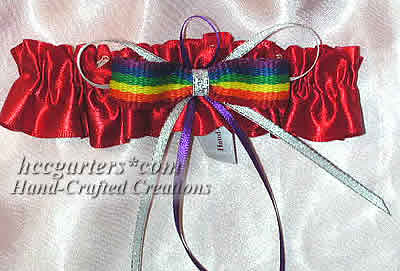The image features a colorful wristband or headband prominently displayed against a satiny white cloth background. At the center of the red elastic band, a bow has been meticulously tied, incorporating multicolored ribbons in hues of red, orange, yellow, green, blue, and purple, accentuated by a small purple ribbon and a silver crystal-like bow. An overlay text towards the bottom left center of the image reads "licegarters.com" followed by "handcrafted creations." The well-lit photograph, likely taken indoors in a store or for an online listing, showcases the new and vibrant quality of this handcrafted piece, designed to catch the eye with its vivid colors and intricate detailing.